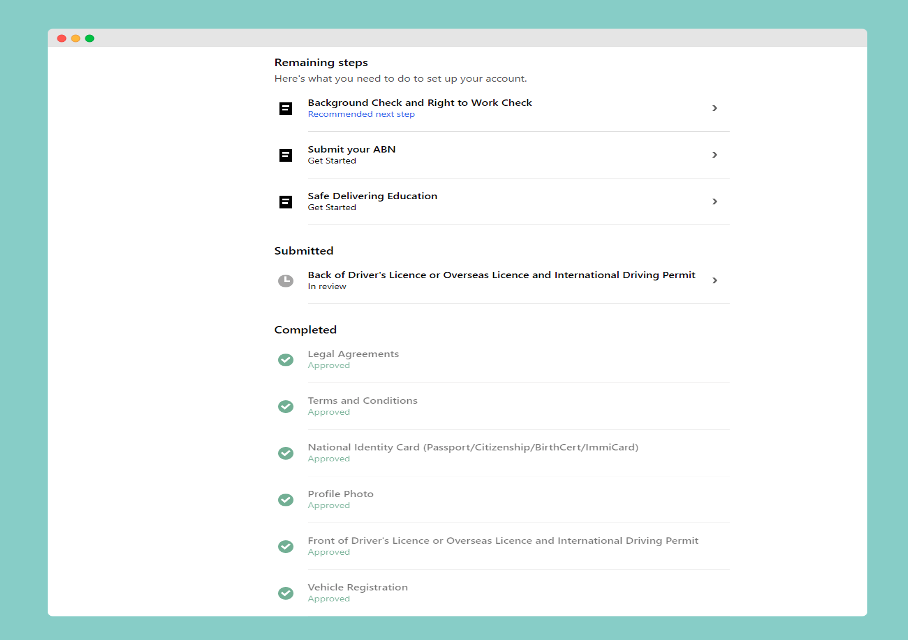The image depicts an Apple-style interface window. In the top-left corner, there are three iconic circles: one red, one yellow-orange, and one green, possibly representing window control buttons. The window itself has a clean, white background with black text, formatted to be center-justified.

At the top center, the text reads "Remaining Steps," which serves as a heading indicating instructions to complete account setup. Listed below are three items in a bold, black font, each indicating a task with a right-aligned arrow suggesting a dropdown option. The tasks are: 
1. Background Check and Right-to-Work Check.
2. Submit your ABN (Australian Business Number).
3. Safe Delivery and Education. Each item has a "Get Started" prompt next to it with an arrow for further actions.

Beneath these tasks, there is a section labeled "Submitted." It lists "Back of Driver's License or Overseas License, International Driving Permit." An adjacent clock icon and "In Review" label suggest that this submission is currently being processed.

Finally, the bottom section, titled "Completed," includes various tasks marked with check marks and displayed in a grayed-out font, indicating they have been successfully finished.

Overall, the layout is clean and intuitive, guiding the user through the necessary steps to complete their account setup.